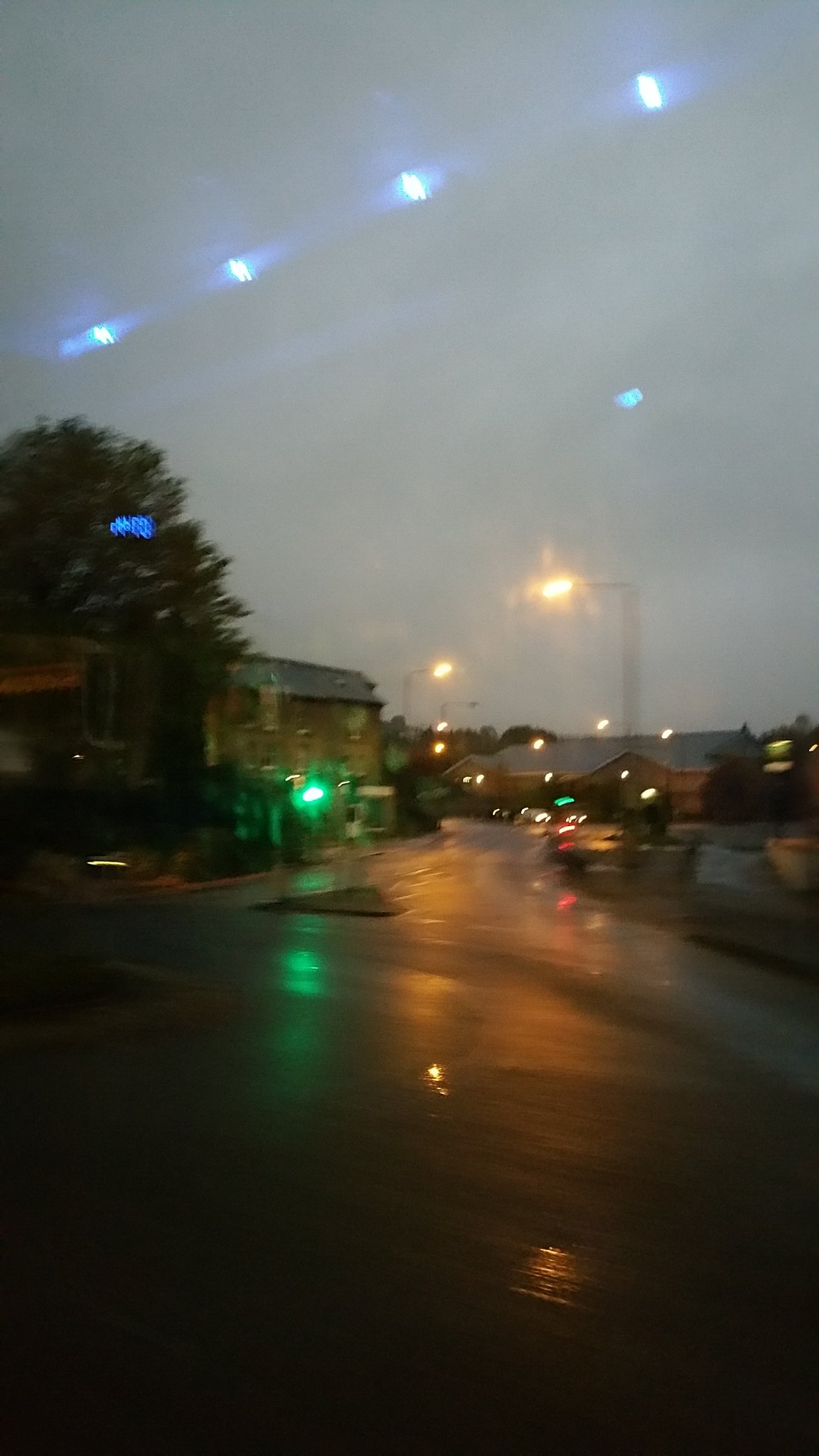This color photograph captures a blurry street scene at the break of dawn or the onset of dusk. The sky is a muted grey, casting a somber mood over the scene. In the sky, four round, bluish lights, potentially reflections, appear almost like hovering UFOs due to their disembodied and surreal nature. Just below these lights lies a smaller, similarly colored light. The scene suggests the photograph was taken through a glass window, given the reflective quality of the lights.

The bottom half of the image is dominated by a dark road, which reflects the green glow of a traffic light positioned centrally in the photograph. Additional reflections of street lights add to the moody ambiance. To the left, the silhouette of a large tree can be seen, beside which stands a tall building characterized by a grey roof and brown walls. Beyond the street lights, several buildings fade into the background, their presence softened by the dim lighting. Overall, the scene feels ethereal, with various light sources and reflections blending to create a mysterious, almost otherworldly atmosphere.